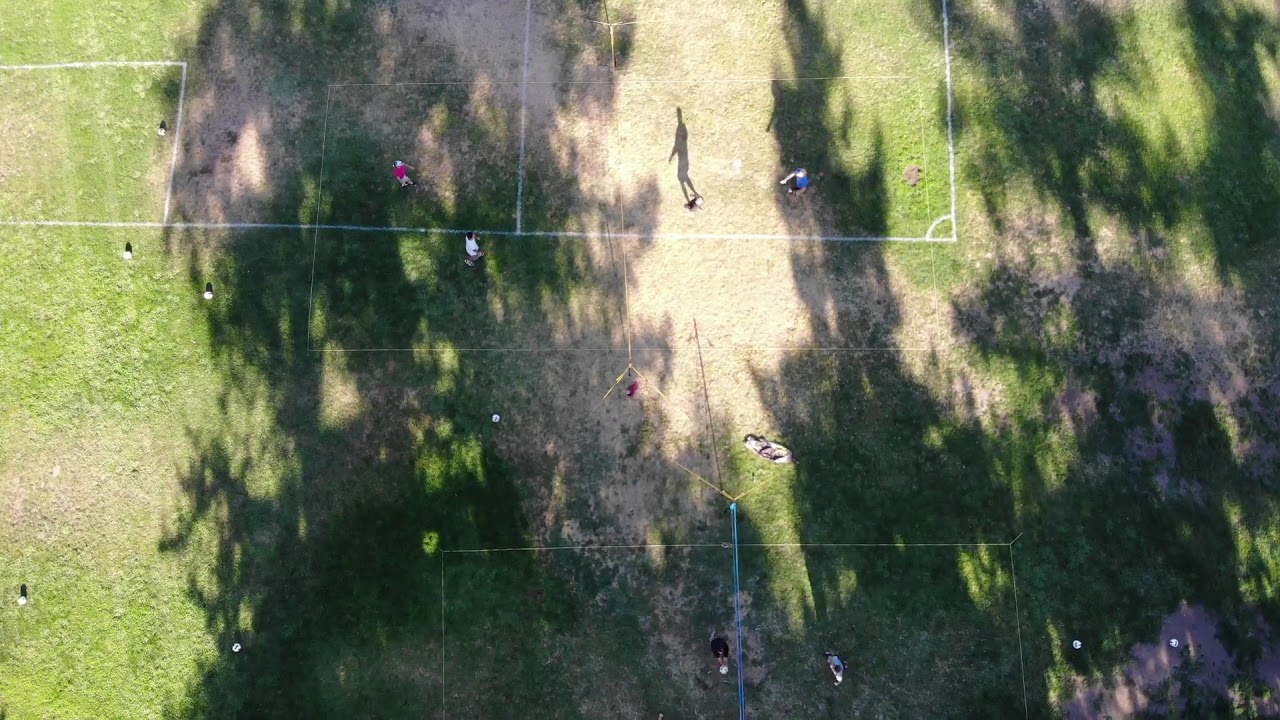This aerial photograph captures a group of people scattered across a grassy field on a sunny day. The field varies in color with green grass interspersed with patchy brown spots. The scene is marked by several white and yellow lines, possibly for sport or surveying purposes, including rectangular and triangular shapes. Among the figures, there's an elongated silhouette of a man prominently positioned in the bright center of the image. Additionally, shadows from three trees are visible, adding depth to the landscape. The photo, which lacks text, also features scattered small white dots or balls, hinting at some outdoor activity. Despite the image's blurriness and distant perspective, it vividly depicts a day spent outdoors within a detailed and divided grassy field.